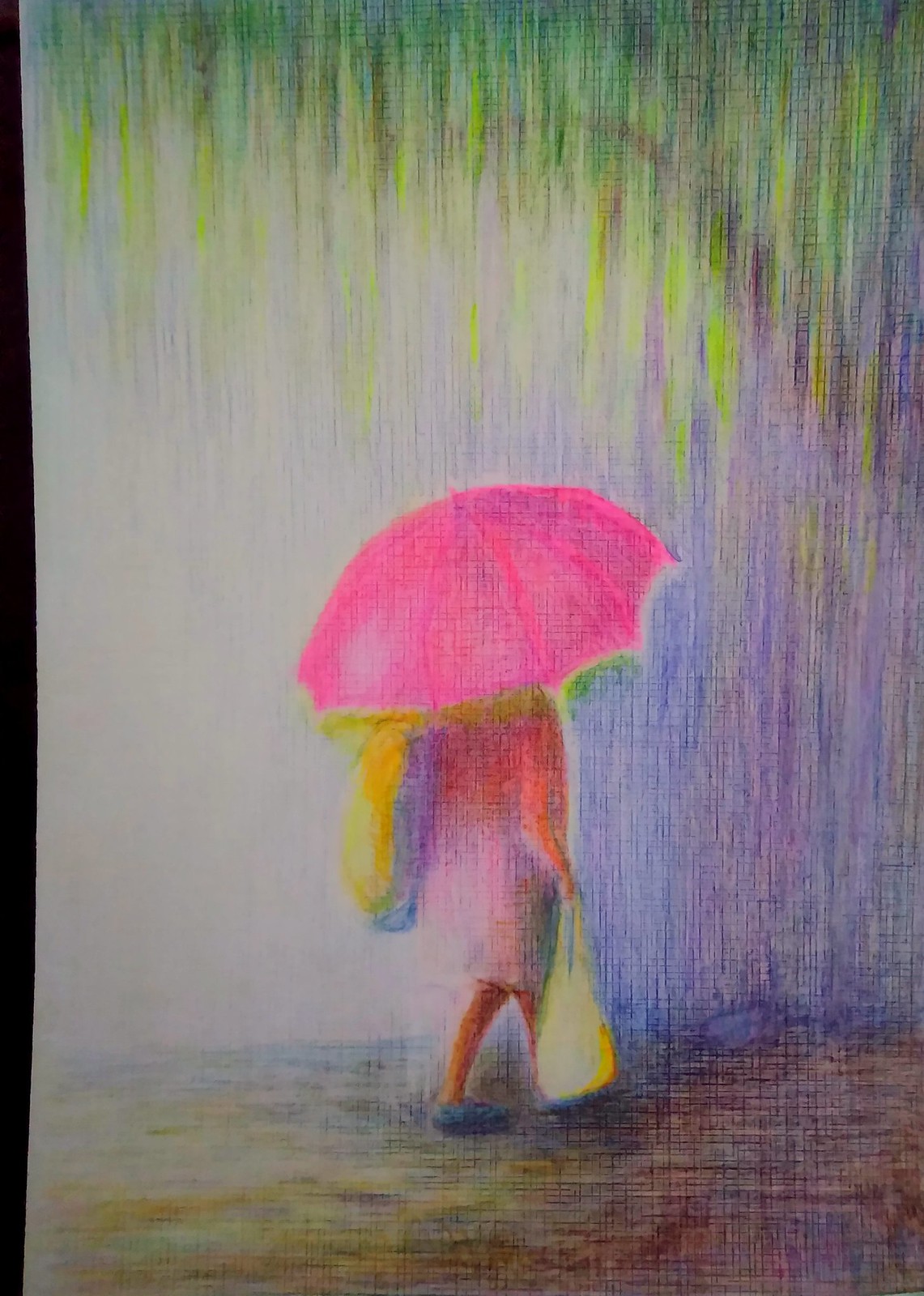In this hand-drawn image, likely created with colored pencils judging by the texture, a blurry yet evocative scene unfolds in vibrant colors. The central figure, seen from behind, is a woman walking towards the right. She carries a hot pink umbrella that contrasts with her pale pink dress. Underneath the umbrella, she wears a long-sleeve red shirt paired with a purple skirt and blue shoes. Slung over her left shoulder is a yellow and purple bag, and she holds a white plastic bag in her right hand. The ground beneath her is a mix of brown, yellow, and purple hues, suggesting a sidewalk or path during a multicolored rainstorm. To the right, a tree with a purple-tinted trunk stands against a white background. The scene is framed by green and yellow rain descending from a blue sky, adding a surreal atmosphere to the picture. There is no text in the image.